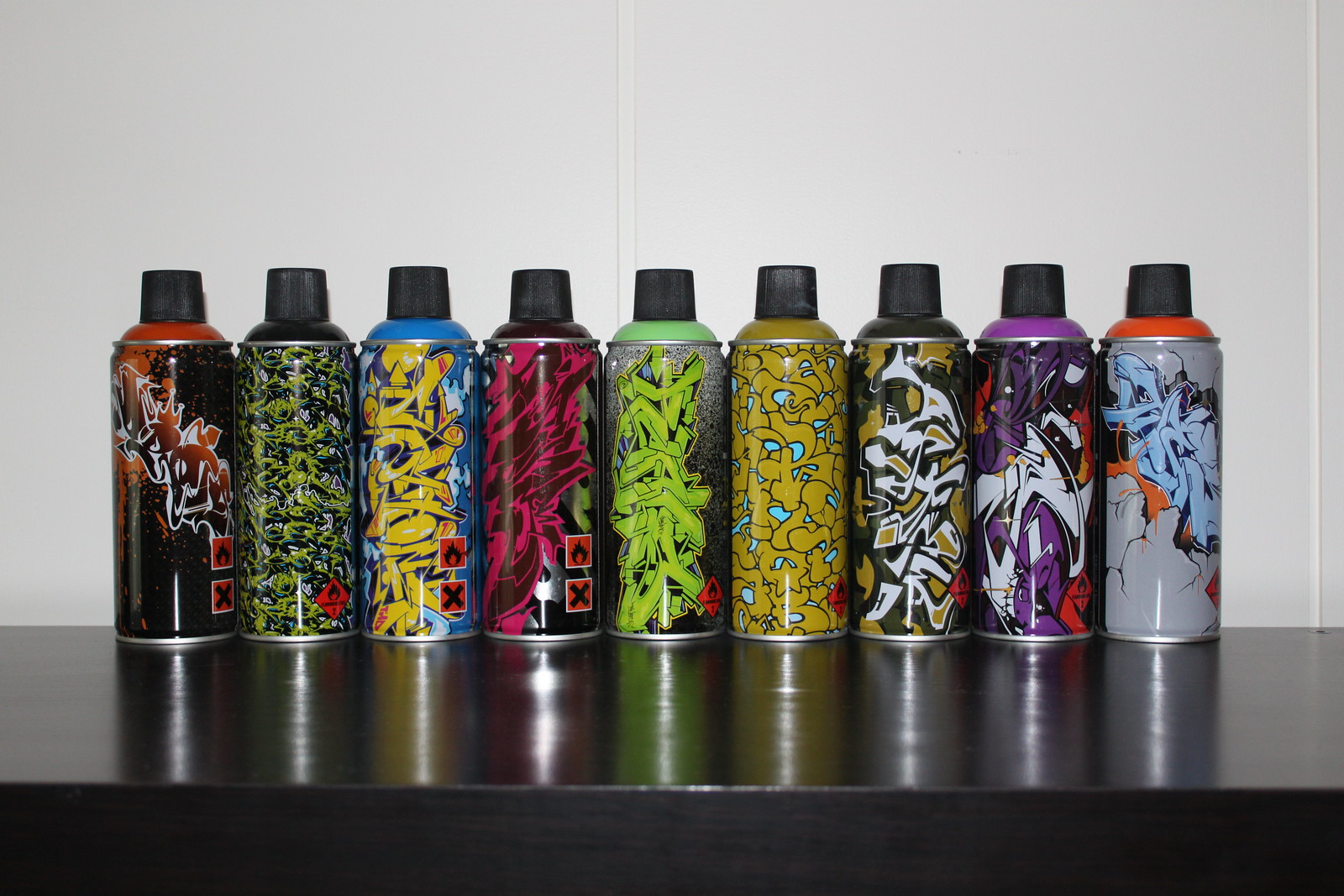In this vivid photograph, nine spray paint cans are neatly aligned in a row on the edge of a sleek black table, set against a stark white wall. Each can is adorned with unique graffiti-style designs featuring a burst of colors, showcasing the variety of hues suitable for street art. The cans, each capped in black, range in color combinations: the leftmost can is adorned in black and orange, followed by one in green, white, and black. The next can boasts yellow, orange, and blue, while the subsequent cans display vivid patterns in pink, green, black, mustard, blue, purple, white, red, blue, gray, and orange. Their position on the table creates a reflective effect, emphasizing their vibrant, rebellious spirit. Each can, decorated with distinct graffiti logos, is a testament to the diverse palette and style options available for graffiti artists.